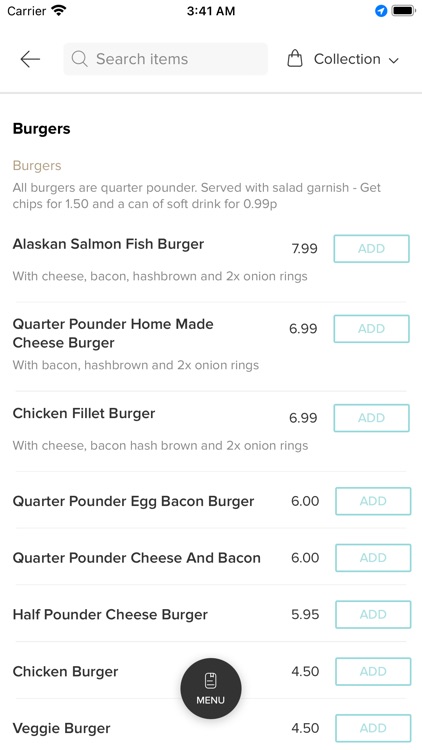Here is a refined, detailed caption for the image:

---

Screenshot of a mobile website interface displaying a menu for a burger restaurant. The interface has a white background with black text at the top indicating the carrier name and full cell phone service. The current time displayed is 1:43:41 AM. To the right, there are blue icons for GPS and a black icon for a fully charged battery.

Below this, there is a navigation section: an arrow pointing to the right, a grey search bar, and a black shopping bag icon with a dropdown. Following this, a section titled "Burgers" in black text has a grey subheading detailing that all burgers are quarter pounders served with a salad garnish. Additional items such as chips for $1.50 and soda for 99p are mentioned.

The menu begins with the following items:
- **Alaskan Salmon Burger, $7.99** - Grey text description: With cheese, bacon, hash brown, and 2x onion rings.
- **Quarter Pounder Homemade Cheeseburger, $6.99** - Grey text description: With bacon, hash brown, and 2x onion rings.
- **Chicken Filet Burger, $6.99** - Grey text description: With cheese, bacon, hash brown, and 2x onion rings.
- **Quarter Pounder Baked Bacon Burger, $6.00**
- **Quarter Pounder Cheese and Bacon, $6.00**
- **Half Pound Quarter Cheeseburger, $5.95**
- **Chicken Burger, $4.50**
- **Veggie Burger, $4.50**

Between the Chicken Burger and Veggie Burger entries, there is a black circle with the words "Menu" and "Wait."

Each burger option on the right-hand side features a grey box with the word "Add" centered in grey text.

---